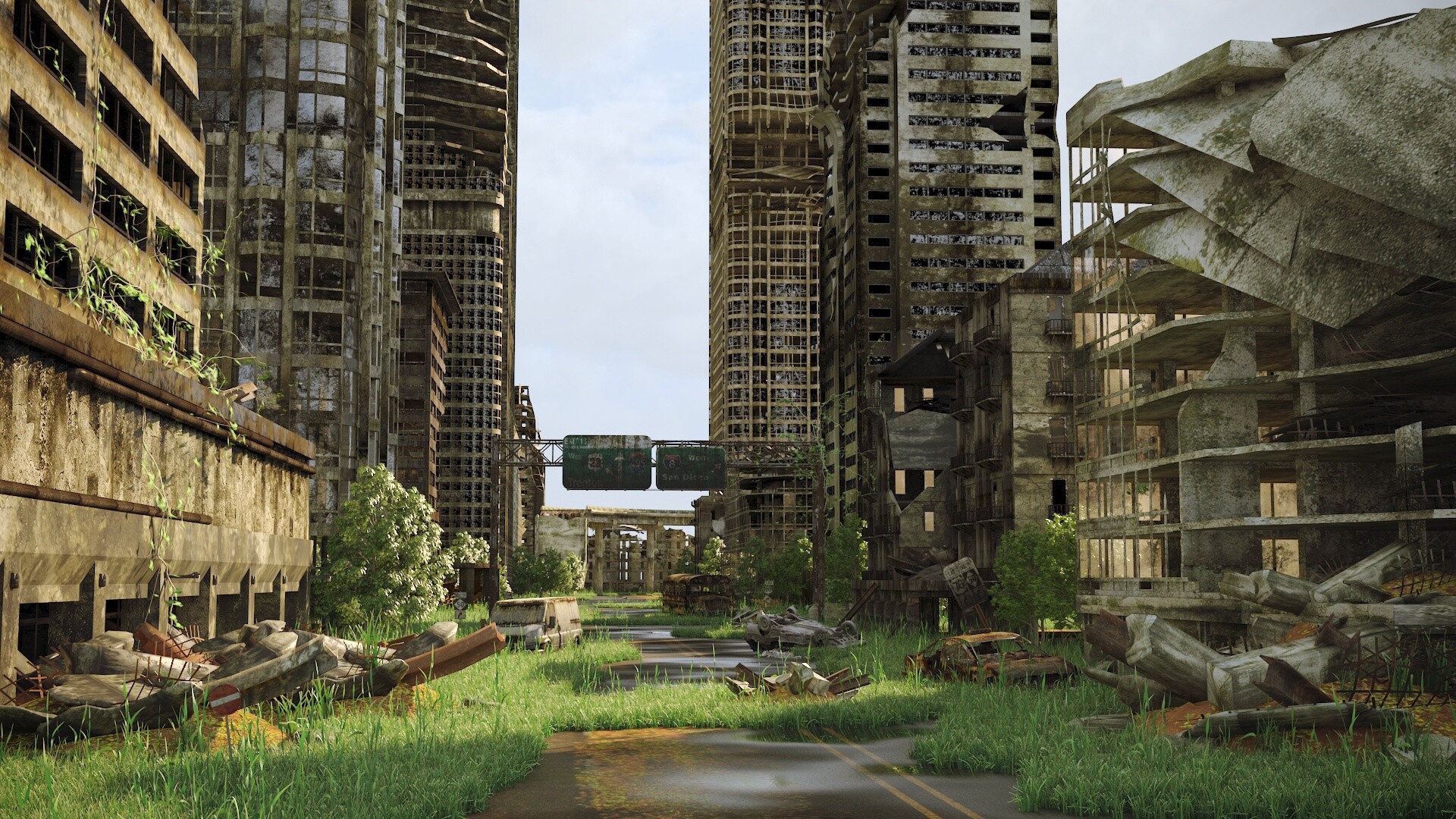The image depicts a haunting, post-apocalyptic scene of an abandoned city that appears to have been reclaimed by nature. Dominating the foreground on the right is a collapsing parking garage, its upper levels caved in, surrounded by rubble. The street itself, identifiable by a faded yellow center line, is overtaken by tufts of grass. Scattered across the road and its shoulders are rusted-out cars and buses, remnants of a time when the city was alive. Flanking the street, dilapidated skyscrapers loom, their dirty facades cracked and crumbling, with shattered windows and overgrown plants clinging to their surfaces. Street signs, battered and weathered, hint at the city’s once functional infrastructure. The overall scene carries a digital or possibly AI-generated feel, with some details blurred, suggesting a combination of artistic elements in portraying what was once a futuristic city now left to decay.